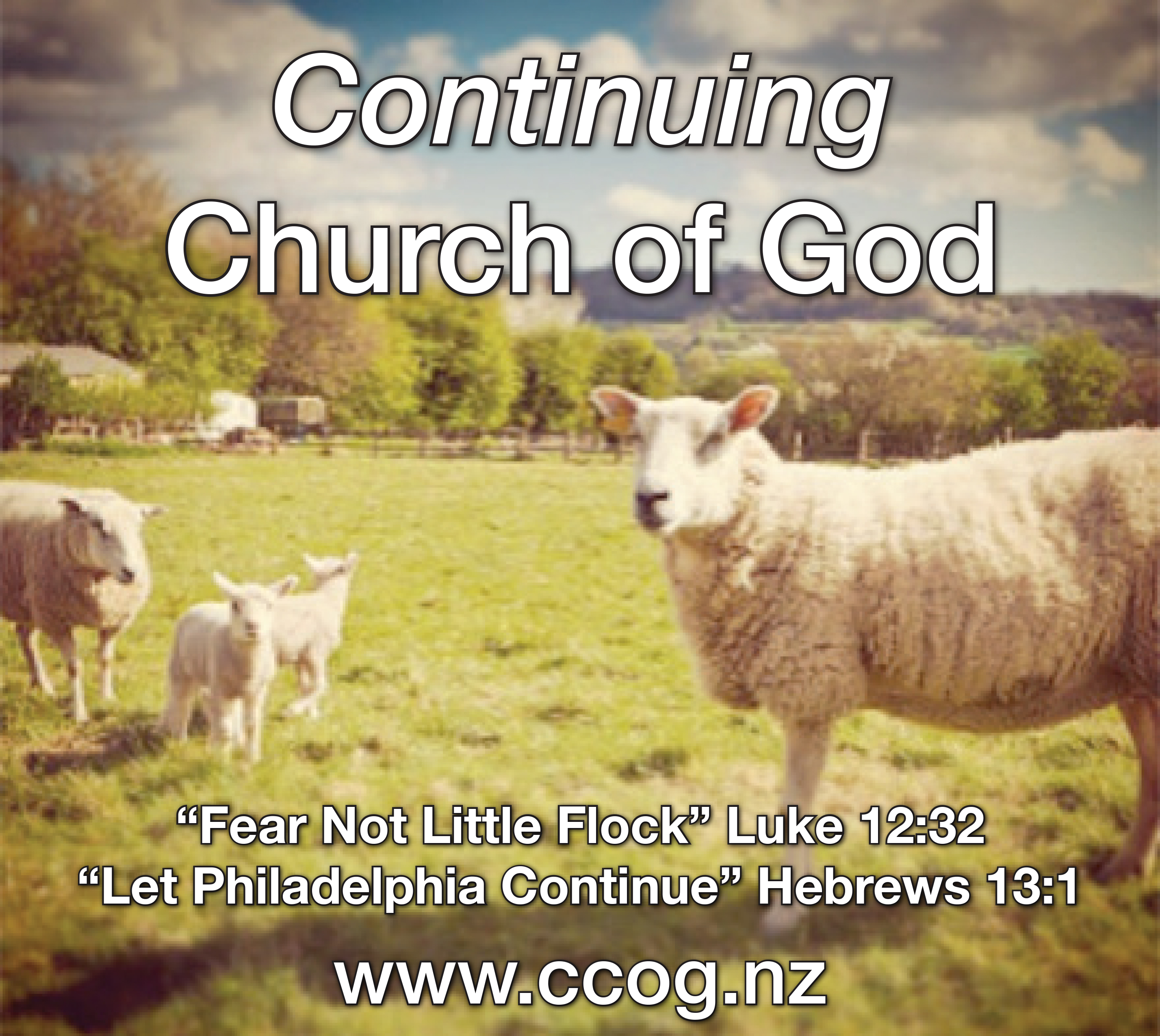The image depicts a serene pastoral scene with four sheep—two adults and two lambs—standing in a lush green field. Among the sheep, the one on the right is facing the camera directly, while on the left, a smaller adult and two cute lambs stand together. The background reveals a rustic wooden fence with a variety of trees behind it, adding to the peaceful rural setting. A small building and a wagon are also visible, contributing to the farm-like atmosphere. Overhead, a vibrant blue sky is dotted with large, fluffy clouds. In large white text with a thin black outline at the top of the image, it says "Continuing Church of God." At the bottom, the text reads, "Fear not, little flock," quoting Luke 12:32. Below that, another quote appears: "Let Philadelphia continue," from Hebrews 13:1. Finally, the website www.ccog.nz is listed at the bottom. The overall scene portrays a tranquil day in a field, reflecting the messaging of comfort and faith conveyed by the accompanying text.